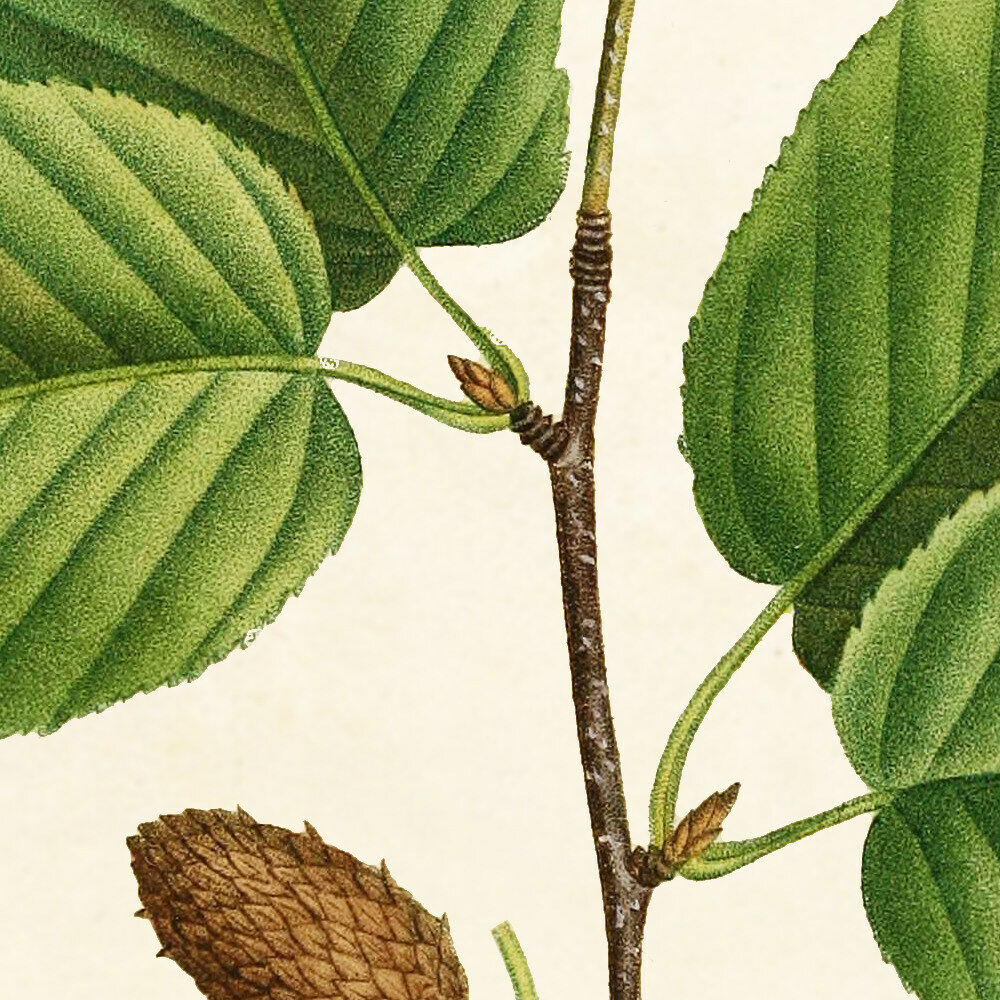This illustration depicts a detailed botanical study with a tall brown stem that transitions to green at the top, set against a faint pale yellow background. The stem features two pairs of green leaves with standard vein patterns, with the top pair sprouting toward the upper left and the bottom pair growing toward the lower right. At the junction where the leaves connect to the stem, there are the beginnings of small buds. Toward the bottom left, attached to a secondary stem, is a larger structure resembling a light brown pine cone, indicative of an unbloomed flower or mature bud. The overall scene presents a close-up, almost jungle-like texture, highlighting the natural growth stages of the plant.